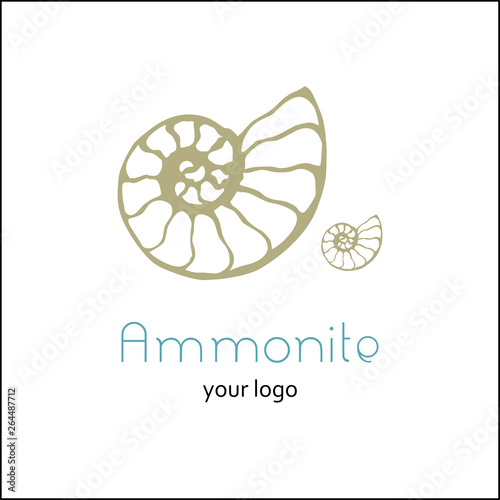The image showcases a detailed portrayal of two conch-like shells intricately spiraled into a swirl formation. The larger shell dominates the composition, with a smaller, precisely mirrored shell positioned to its right. Both shells exude a light gold hue. Beneath the shells, the caption reads "Ammonite" in a refined, delicate teal font, while the phrase "your logo" appears below in lowercase black sans-serif typeface. The entire image is marked with Adobe Stock watermarks, and an additional "Adobe Stock" text is placed in black in the bottom left corner.